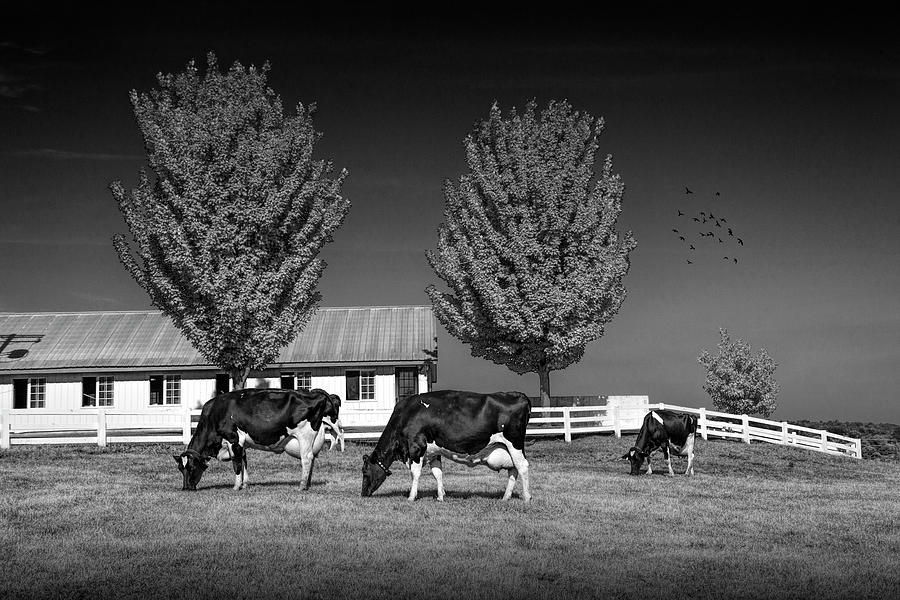This black-and-white photograph captures a tranquil rural scene featuring three black and white cows grazing in a well-kept field. The cows, characterized by their black backs and white legs, are positioned prominently in the center of the image, with their heads down as they munch on the grass, which, despite the grayscale, likely appears verdant in color. A white picket fence stands behind them, offering a boundary to the scene.

To the left of the cows, a large white barn with multiple windows and a possible steel roof adds structure to the rustic tableau. The barn's roof and sides are dotted with windows placed at regular intervals, emphasizing the length of the structure. Behind the cows are three trees: two imposing, tall trees providing a canopy of foliage, and a smaller bushier tree enhancing the layered landscape.

The sky above creates a dramatic backdrop with its varying shades of black and gray, typical of black-and-white photography, and it is punctuated by the subtle silhouettes of birds in flight. The overall ambiance of the image is enhanced by a vignette effect, with the edges of the photograph gradually darkening, drawing the viewer’s focus toward the serene pastoral scene in the center.